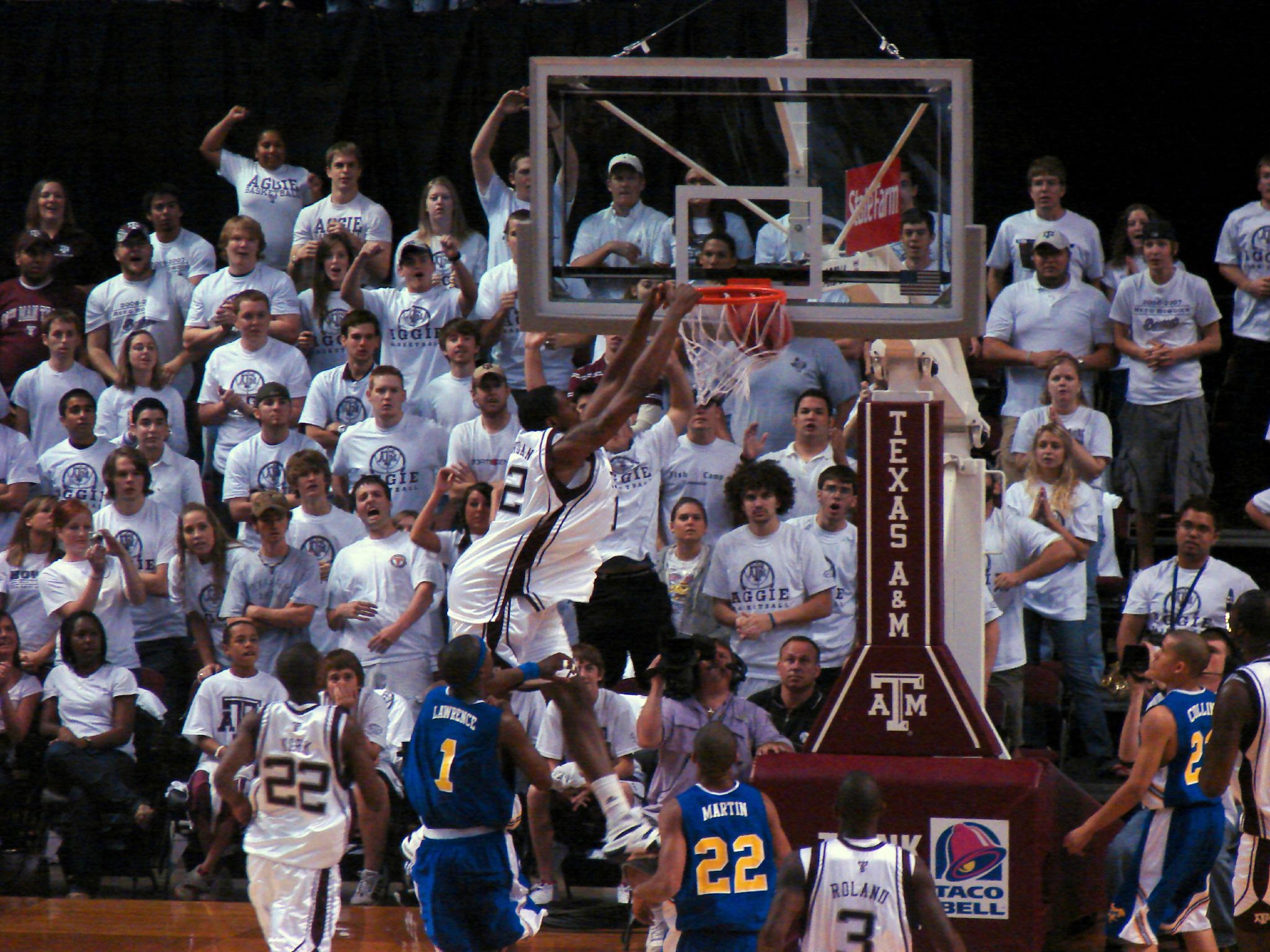In the center of the image, a basketball player is caught in mid-air as he dunks the ball into the hoop, surrounded by the action of a live game. The hardwood flooring of the court reflects the intensity of the moment, adding a polished sheen to the scene. At the top of the image, a crowd of spectators, a mix of those seated and standing, focus intently on the thrilling play. The hoop prominently displays the text "Texas A&M," hinting at the location or team involved in the game. Nearby, a Taco Bell sponsorship is faintly visible, suggesting commercial partnerships. The color palette of the image is rich and varied, including shades of black, white, maroon, brown, blue, yellow, gray, and red. The setting is an indoor basketball arena filled with daytime light, emphasizing the lively atmosphere of the game.